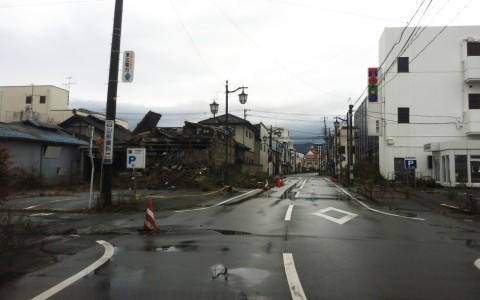The photograph captures a dimly lit, overcast street at an intersection in an older part of a city, characterized by its worn and somewhat dilapidated buildings. The wet pavement, marked by puddles, indicates that it has recently rained. The street is lined with two- and three-story buildings, some of which appear to be partially collapsed or in disrepair, adding to the scene's aged and somewhat neglected atmosphere. Streetlights and telephone wires run along the road, which is a two-lane highway with white markers indicating the middle of the road. Orange traffic cones are placed conspicuously in the street, particularly at one entrance, suggesting ongoing construction or obstruction. The area appears deserted, with no people or cars visible, enhancing the impression of an abandoned or quiet moment in an otherwise busy urban setting. The lack of greenery and the cloudy sky contribute to the overall gray, muted tone of the scene.